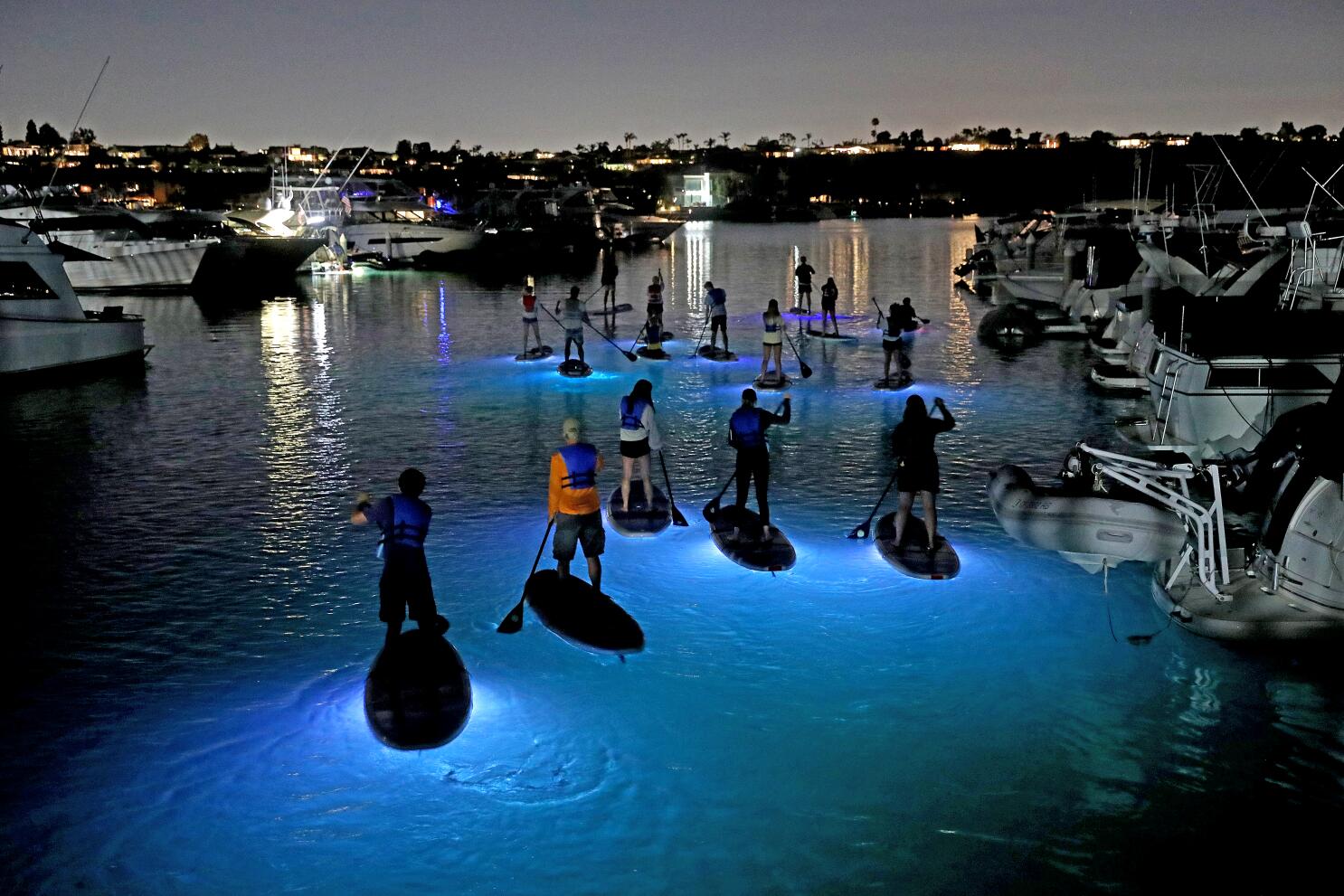In this striking nighttime photo taken at a marina, a large group of roughly a dozen people is seen paddleboarding on the glowing water. The enchanting blue light illuminates the water beneath their paddleboards, creating a vibrant, eye-catching effect that turns the scene into an ethereal spectacle. The paddleboarders, silhouetted against the dark sky, are equipped with long paddles and are notable for their colorful attire, including blue life vests, white clothing, and flashes of orange shirts. Surrounding the paddleboarders, boats are visible on both sides of the marina, further enhancing the bustling atmosphere. The dark background, dotted with trees and the dim, gray sky, adds to the photograph’s overall nocturnal charm and serene ambiance.